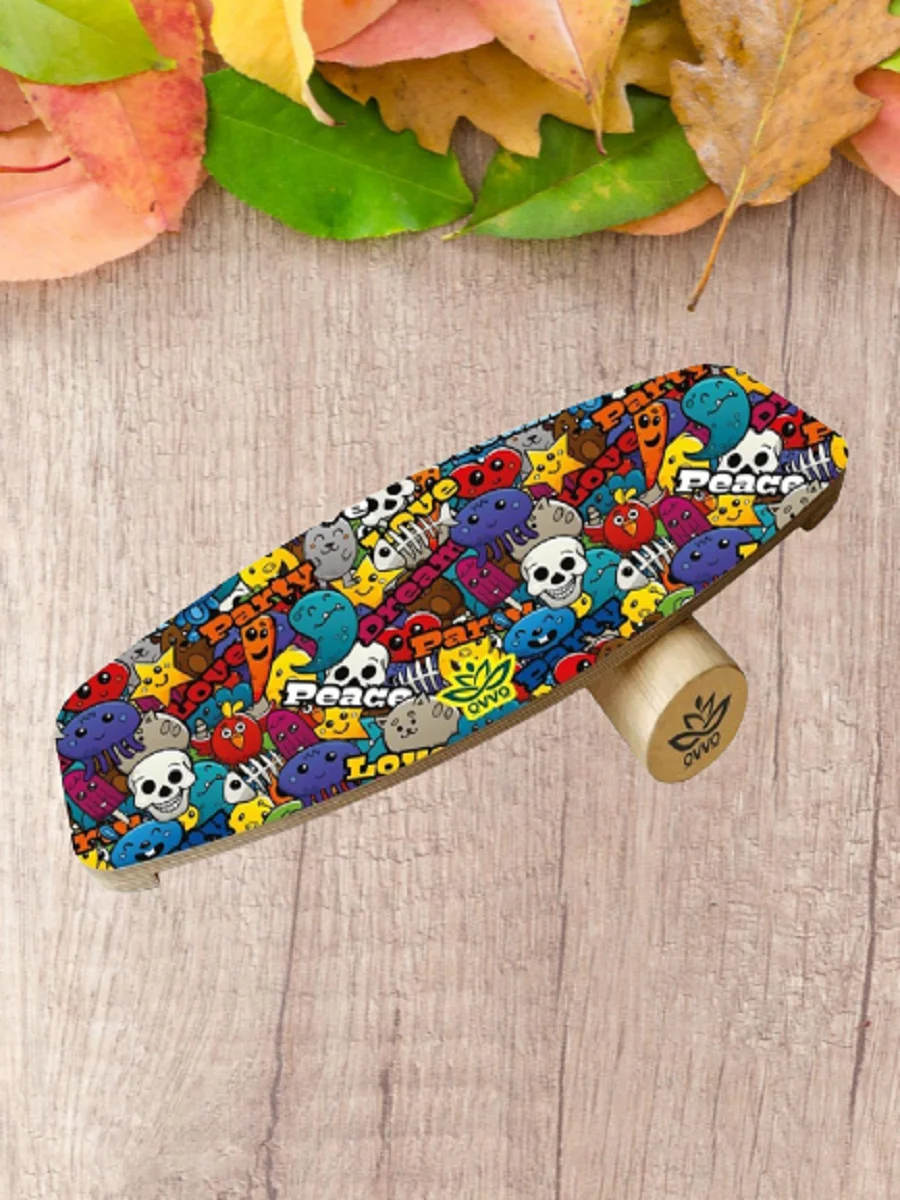This detailed image features a surreal photograph that appears to be digitally manipulated, showcasing a balance board propped against a cylindrical wooden peg amidst a wooden backdrop. The balance board, with its skateboard-like shape, is adorned with vibrant and whimsical graphic designs including little monsters, animals, a skeleton head, a jellyfish, and a star. The colorful palette consists of blue, white, yellow, orange, red, and green hues that bring the illustrations to life. Interspersed among the drawings are the words "love," "party," "dream," and "peace" in various bright colors. The wooden cylinder that supports the board has a light beige hue with a black symbol of a blooming flower and the inscription "O V V o" below it. The background is composed of pale wood, with random leaves scattered at the top of the image in green, yellow, and orange, contributing to the overall autumnal feel. The leaves seem disproportionately large compared to the board, adding to the collage-like, photoshopped appearance of the image. The balance board itself appears to float ambiguously in the composition, enhancing the dreamlike quality of the scene.